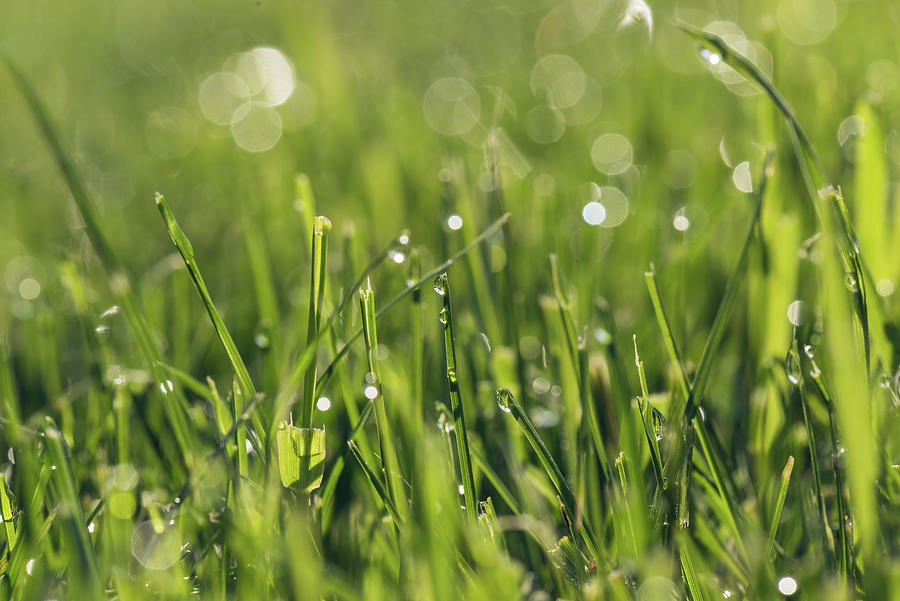This close-up image captures the vibrant, lush green blades of freshly cut grass, likely in a lawn. The scene appears to be illuminated by sunlight, adding a bright and lively quality to the grass. Each blade is accented with large, glistening water droplets, perhaps indicating morning dew or recent rainfall. The water droplets refract light, creating a shimmering effect, and through them, the surrounding grass appears beautifully distorted. Some of these water droplets contribute to a bokeh effect, presenting as semi-transparent white circles in the blurred background. Among the predominantly green grass, a few light yellow leaves are discernible, adding subtle contrast. The photograph also includes some translucent circles towards the top, possibly lens flare or camera artifacts, adding to the ethereal quality of the image. Overall, the play of light, dew, and the lush grass combined create a refreshing and dynamic scene.